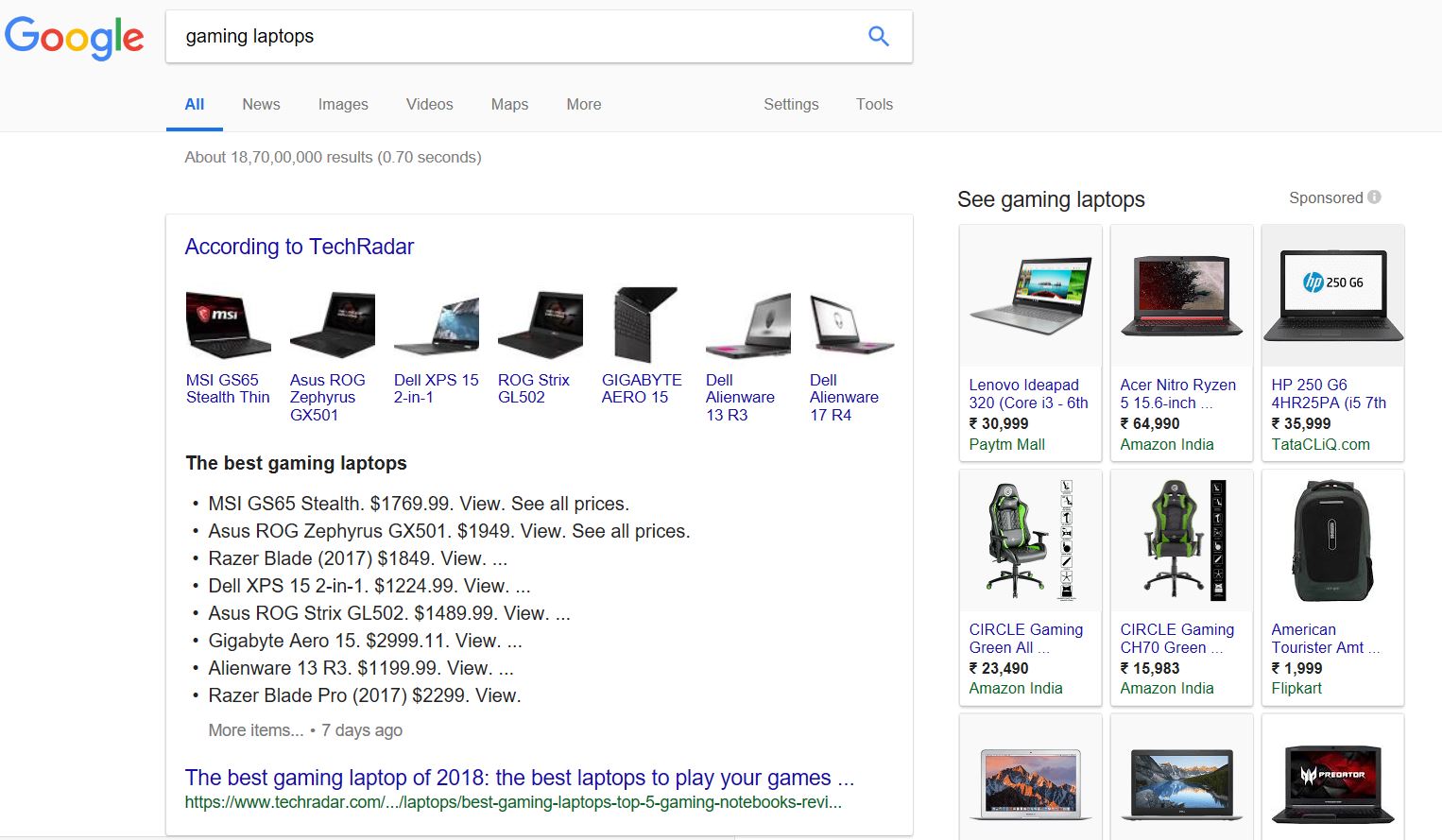A detailed screenshot from a Google search result page for "gaming laptops". The familiar Google logo is prominently displayed in the upper-left corner, with the word "All" highlighted in blue, indicating the current search category. Beside "All", the search categories "News," "Images," "Videos," "Maps," and "More" are visible, followed by options for "Settings" and "Tools" on the right. Below these, the number of search results and the time it took to retrieve them are noted.

In the search results, an excerpt from TechRadar is displayed, along with images of various gaming laptops. The highlighted models include the MSI GS65 Stealth Thin, the Asus ROG Zephyrus GX501, a Dell laptop, an Asus Strix model, and the Gigabyte Aero, among others. A section labeled "The best gaming laptops" features a detailed listing starting with the MSI GS65 Stealth Thin priced at $1,769.99. Accompanying this are articles such as "The Best Gaming Laptops of 2018" and "The Best Laptops to Play Your Games," with corresponding images on the right side of the screen.